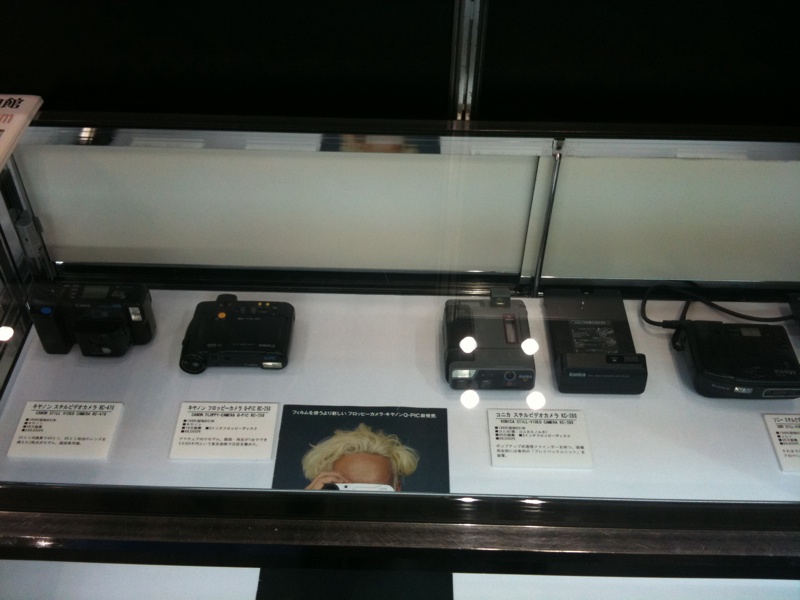This color photograph, taken in landscape orientation indoors, showcases a meticulously arranged display case. The case itself is constructed with glass panels on the top and sides, a white back, and is rimmed with dark brown wood. Inside, the display features various pieces of electronic equipment, prominently including several black cameras and what might be pagers or other devices. 

In front of each item are white cue cards with black Japanese text, likely providing information about the objects. At the center of the case, a brochure with a dark blue background and white Japanese text at the top catches the eye. This brochure features the top portion of a man's head with frilly blonde hair and an olive complexion, holding something up to his eyes with his left hand.

The equipment is arranged on a white linen-lined box. Notable items include a standing camera with a blue button on the left and a silver rectangular viewfinder on the right. Another device, lying flat, resembles binoculars with orange buttons on top. There is also a gray object that looks like a tape recorder, identifiable by a red-outlined viewing area for the tape and an earphone jack. Another thin, rectangular item might be a flash or camera, and lastly, a flat rectangular device labeled "Sony" with a silver rectangle for the light and a black rectangle on the front, could be a viewfinder. The display is well-organized, with the lid of the case tilted upward to clearly showcase the items within.